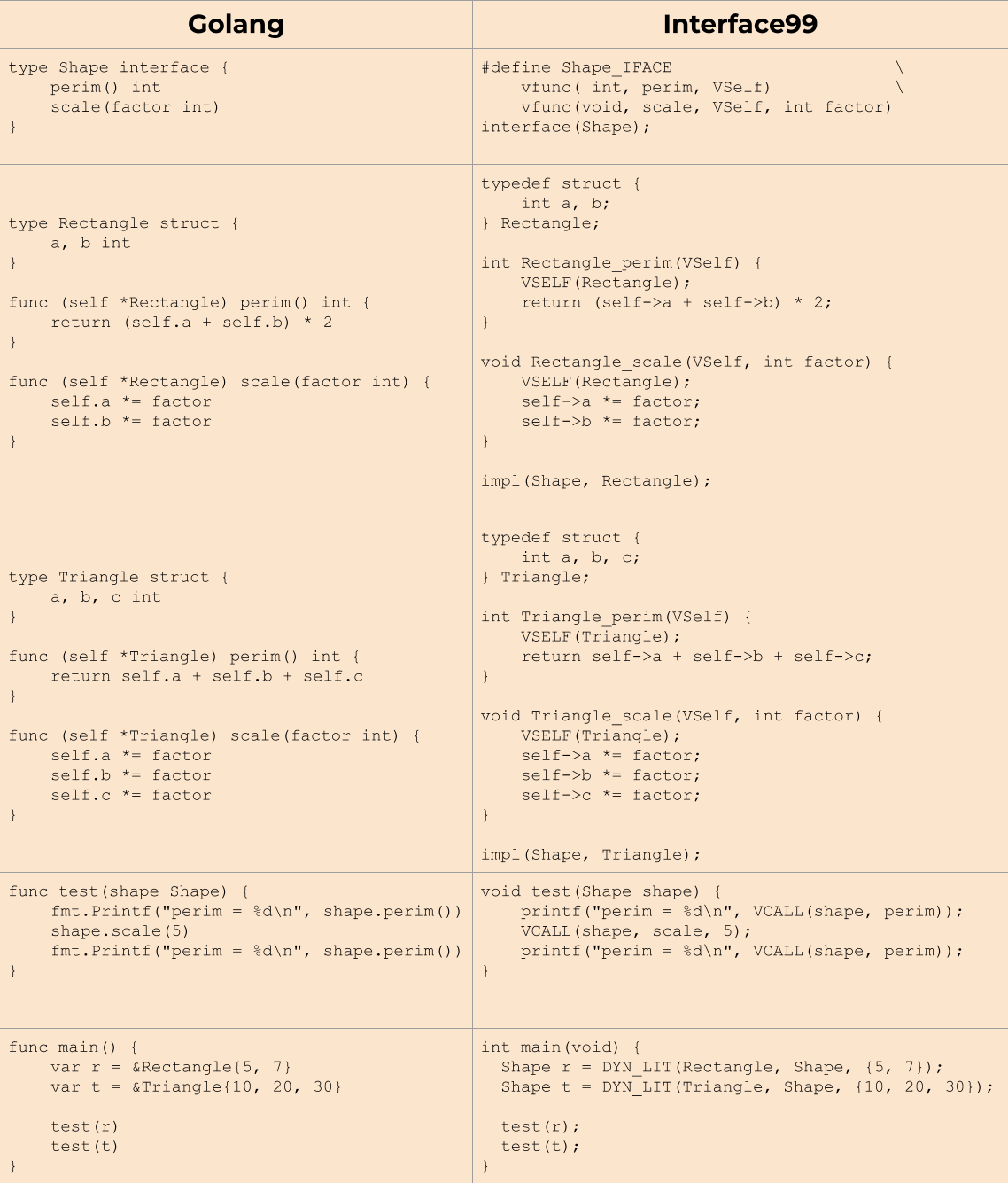A rectangular photo depicting a computer screen is centered on light pink-tan paper. The screen itself is split into ten equal squares, five on the left and five on the right. In the top-left corner of the image, the word "Golang" is prominently displayed in bold black letters, while the top-right corner features "Interface 99," also in bold black letters.

The image showcases a detailed snippet of a computer program, likely written in the Go programming language, focusing on defining various shapes. The left half of the screen contains code segments such as:

- `type Shape interface{}` 
- `type Rect struct { a, b int }`
- `func (r Rect) Area() int { return r.a * r.b }`

Further down, the code expands on these definitions and includes additional constructs like:

- `type Rect struct { A, B int }`
- `func (t Triangle) Area() int { return (t.A * t.B) / 2 }`
  
On the right side of the screen, the programs define interfaces and functions, such as:

- `const PI = 3.14`
- `func main() { r := Rect{2, 3}; t := Triangle{4, 5} }`
- `fmt.Println("Area of Rect:", r.Area())`
- `fmt.Println("Area of Triangle:", t.Area())`

Overall, the program systematically defines several geometric shapes, including rectangles and triangles, while providing methods to compute their areas. The meticulously-organized and annotated code serves as a clear, comprehensive example of object-oriented programming in Go, focusing on functional definitions and interface implementations.